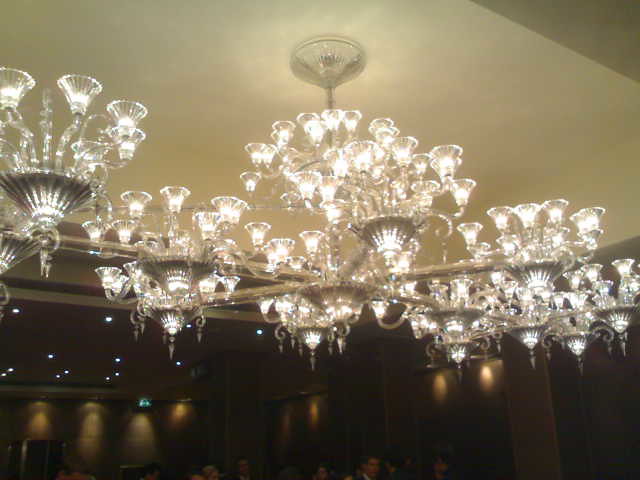This photograph captures a large and intricate chandelier suspended from the ceiling, giving an upward perspective of its grand design. The chandelier features a central silver cap on a white ceiling, from which a silver post descends. Extending from the post are five to six silver bars arranged in a star pattern, each adorned with clear glass flower cups. From these cups, more clear glass arms rise, each culminating in smaller glass flower cups. Every cup is illuminated by white lights, with an estimated total of around 120 lights casting a radiant glow.

The chandelier is decorated with an array of crystal lanterns, light bulbs, charms, and gems, adding to its elegance. The surrounding ambience is predominantly dark, highlighting the chandelier's brilliance. The setting appears to be an opulent restaurant or a hotel event hall, suggested by the dining tables and people seated beneath the chandelier, as well as the surrounding windows. Through one of the windows, there seems to be a view of a small body of water, hinting at a picturesque location. The overall scene exudes sophistication and elegance, characterized by the chandelier's dazzling presence.